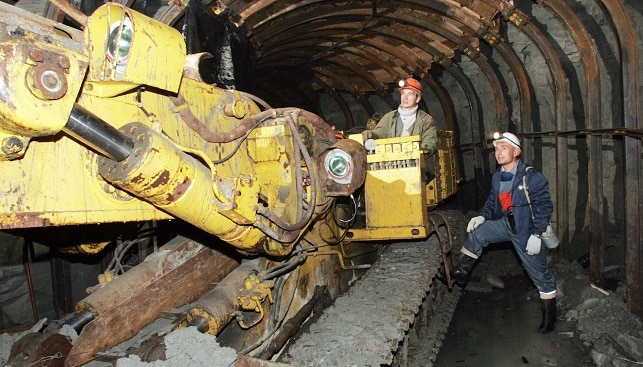In the detailed photograph, two men are working in an underground tunnel, surrounded by a series of metal, brown, arching supports that frame the gray rock interior. The tunnel environment appears wet, with muddy and rusty surfaces on both the machinery and infrastructure. The men are positioned on and around a large, well-worn yellow machine with tank tracks and a prominent piston, suggesting heavy use in excavation or construction. The man operating the machine is dressed in a tan outfit with a brown jacket, a white turtleneck, and an orange helmet equipped with a flashlight. Seated in the driver's seat, he navigates the machinery through the tunnel. Meanwhile, another man, dressed in blue with black boots and white gloves, stands beside the machine with one foot on the tracks. He too wears a helmet with an attached light. Above them, the curved metal beams that support the tunnel appear dirty and corroded, adding to the gritty and industrious atmosphere of the scene.